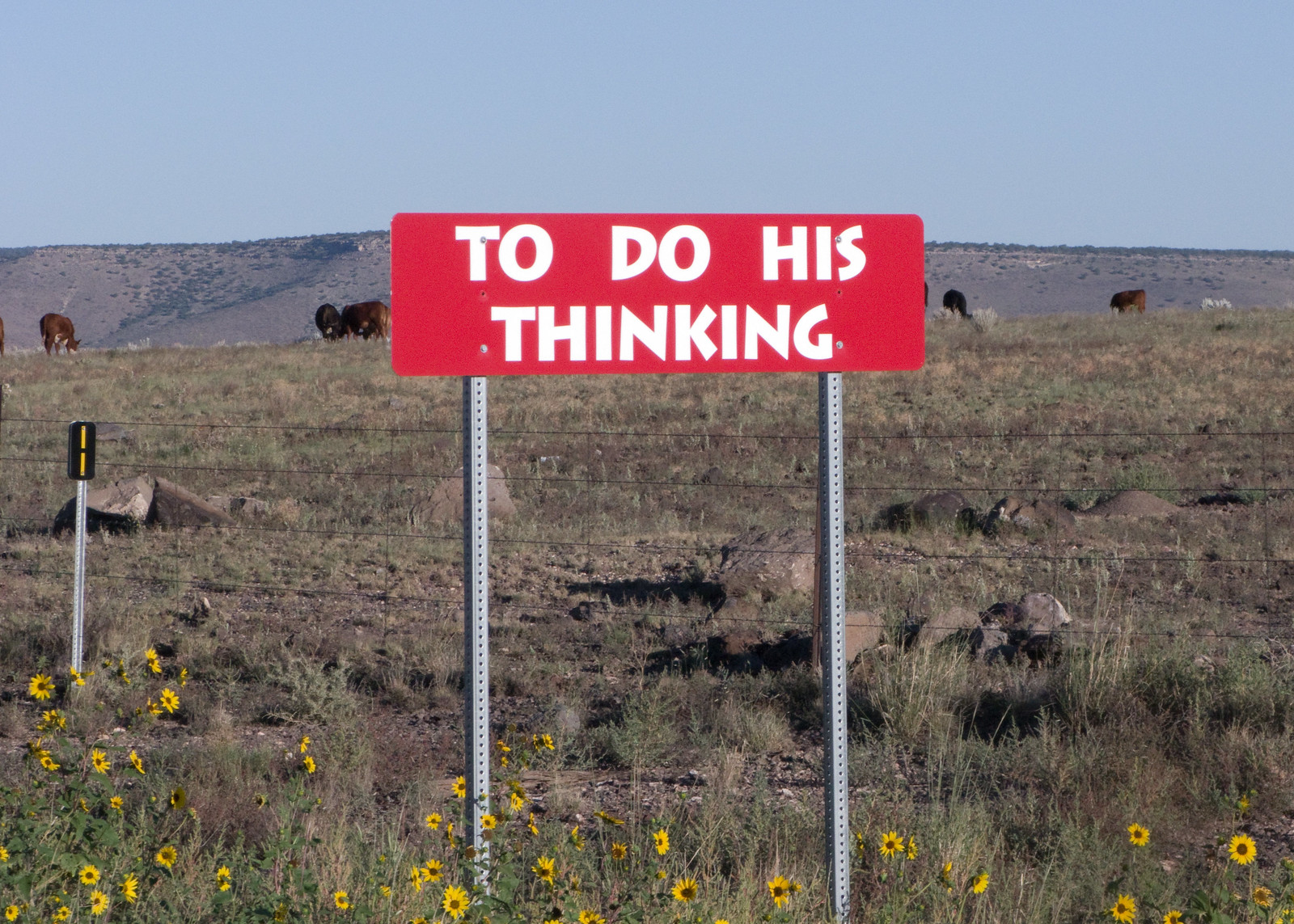On a bright, sunny day under a clear blue sky, a charming semi-arid landscape unfolds. In the foreground, rocky terrain interspersed with patches of brown grass hosts a colorful array of daisies. Their cheerful blooms contrast beautifully with the rugged land. Standing out against this natural backdrop, a prominent billboard is elevated on two silver metal poles. The billboard features a bold red, rectangular background, with the phrase "To Do His Thinking" emblazoned across it in thick white letters. In the distance, the scene transitions to rolling hills and majestic mountains. Grazing serenely amidst this picturesque environment are several brown cows, completing the tranquil and idyllic setting.